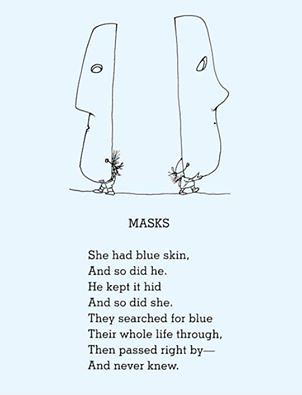This image appears to be a poster featuring a Shel Silverstein poem titled "Masks." At the top of the poster, there is an illustration of a mask being torn apart, held by what seems to be human figures. The poster's color scheme is limited to light blue and black. Below the image of the masks, towards the bottom of the poster, is the poem's text. The poem reads: "She had blue skin and so did he. He kept it hid and so did she. They searched for blue their whole life through, then passed right by and never knew." The overall design and elements suggest a stylized graphic intended to convey an informational or artistic message.